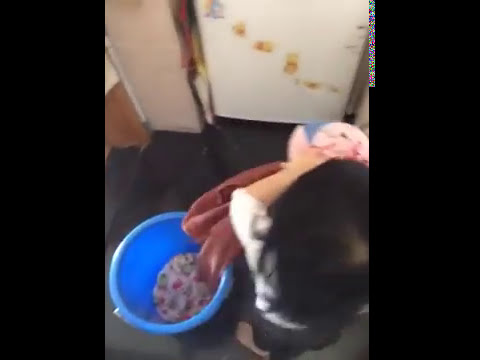The blurry image, taken from above, captures a small kitchen area with a black floor and beige walls. At the center of the photo is a small girl with black hair, dressed in a white shirt and black pants, standing in bare feet near a staircase. She is seen pulling clothing out of a blue bucket. A white refrigerator, adorned with stickers that resemble Winnie the Pooh, is positioned near the stairs. The fridge is partially obscured by what appears to be boxes, potentially for recycling or trash. A faint multicolored pixelation runs along the top right, adding to the overall blur and distortion of the photograph.